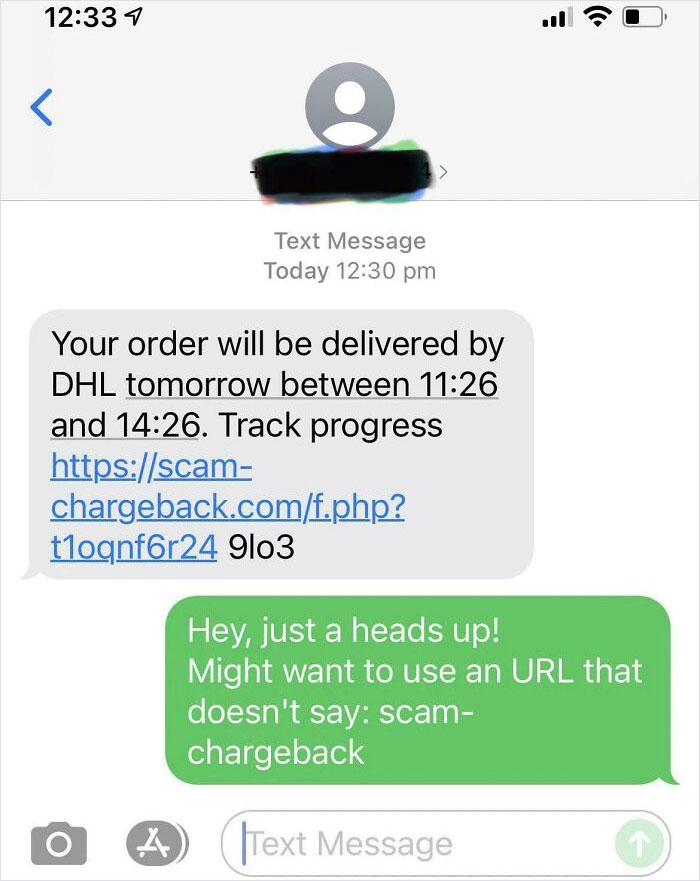Screenshot of a text message conversation from a mobile phone:

The top quarter of the screenshot features a light grey banner. In the top left corner, the time is displayed as 12:33. The top right corner contains icons indicating network connectivity, Wi-Fi usage, and a battery level showing just under 50% remaining. Centered within this banner is a default avatar depicting a white head and shoulders on a darker grey circular background. 

Beneath the avatar, the sender's name is obscured by overlapping blue, red, green, and black marker scribbles. To the left of this area is a blue arrow pointing left. 

Below the banner, the screen displays "Text Message Today 12:30 PM." The text message is enclosed in a light grey speech bubble with rounded edges. The message reads in black text: 

"Your order will be delivered by DHL tomorrow between 11:26 and 14:26. Track progress at [URL: https://scam-chargeback.com/F.php?t10setaqqnf6r24]. 9L03"

Following this, there is a reply in white text on a green background: 

"Hey, just a heads up! Might want to use a URL that doesn't say: scam-chargeback."

Below the conversation, there are icons for a camera and the letter "A" on a darker grey background, along with a text message input box with a blue vertical cursor inside it.